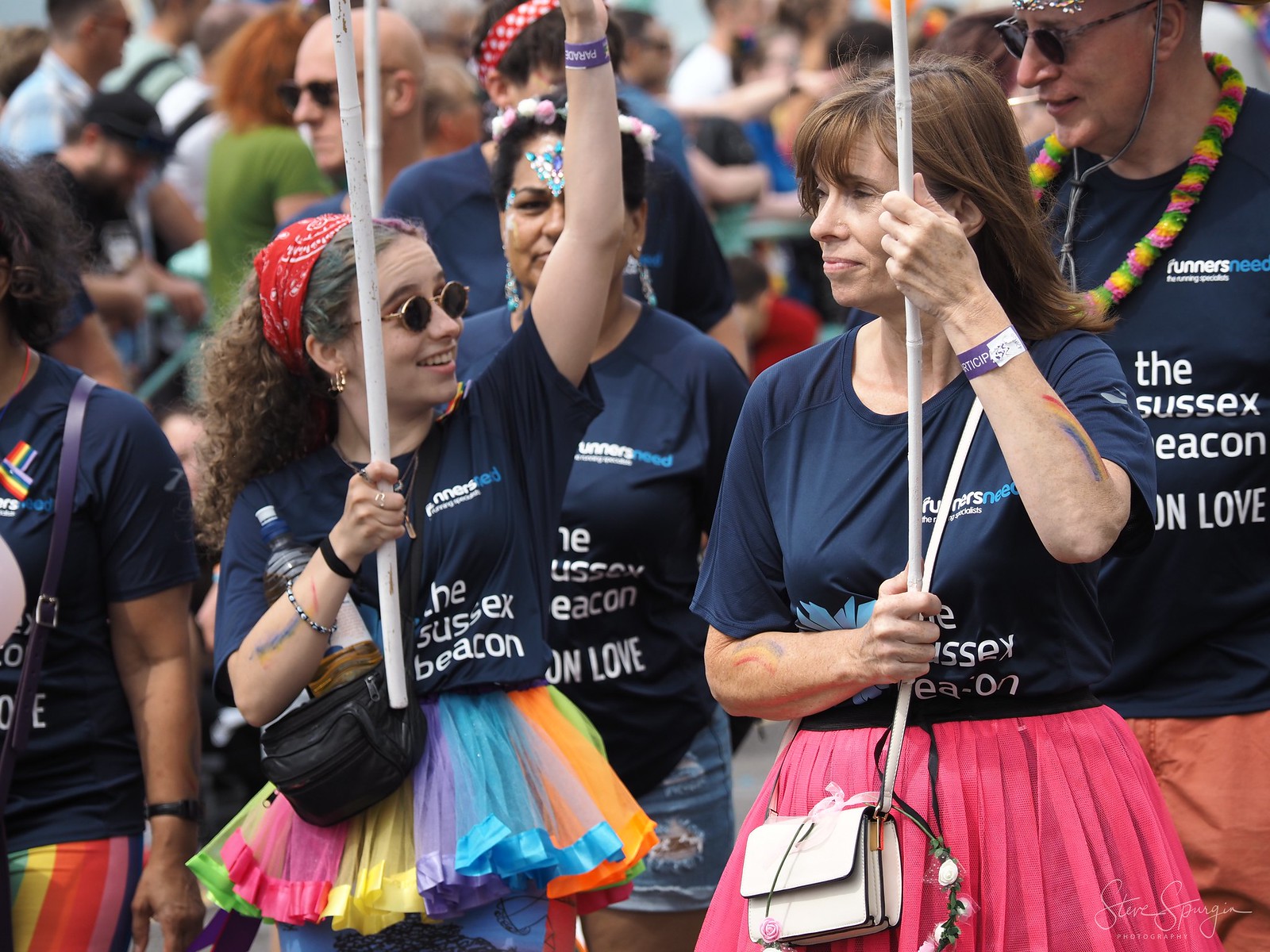The photograph depicts a lively rally or protest, featuring three women prominently in the foreground, each holding a sign, though only the handles of the signs are visible. They are wearing navy blue t-shirts with white text, obscured by their arms and the sign handles. Adding a burst of color, they don distinctive tutus—one pink and another multicolored—over their shirts. Among them, one woman sports sunglasses. The man to the right is adorned with beads around his neck. The crowd behind them, featuring at least six to seven others similarly clad in navy blue t-shirts with partially readable text including "The Sussex" and possibly "Beacon" or "Love," indicates a cohesive group, all participating in the event. The gathering is sizable, with many individuals slightly out of focus, collectively enhancing the bustling and unified atmosphere of this demonstration or march.